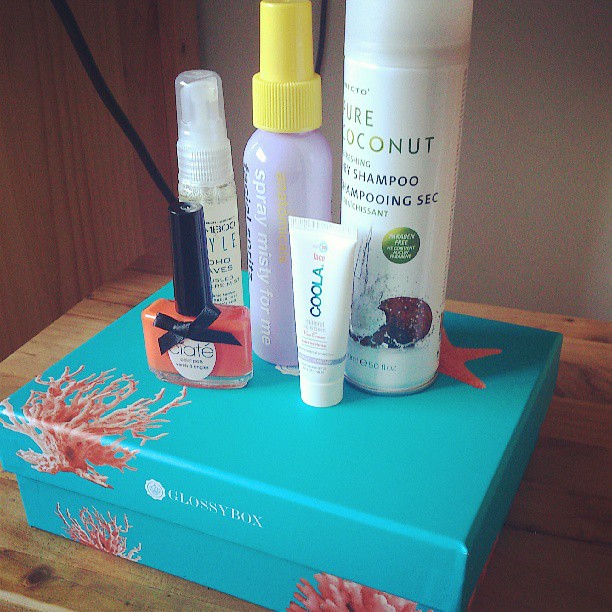The image showcases a collection of beauty products arranged on a light-colored wooden shelf. The focal point is a vibrant, aqua blue subscription box labeled "Glossy Box" in white lettering, adorned with pink coral reef and starfish illustrations. Atop this box are various beauty items: a peach-colored nail polish with a black lid and an adorable black bow, branded "Ciate"; a small white bottle with blue lettering "COOLA" for face lotion; and a larger white bottle labeled "pure coconut dry shampoo," featuring an image of a coconut. Additionally, there's a purple bottle with a yellow cap that reads "Spray Misty for Me." Another bottle behind these items is unreadable. The scene is set against a backdrop of visible cords, a white wall, and part of a wooden wall on the left, completing the indoor setting.